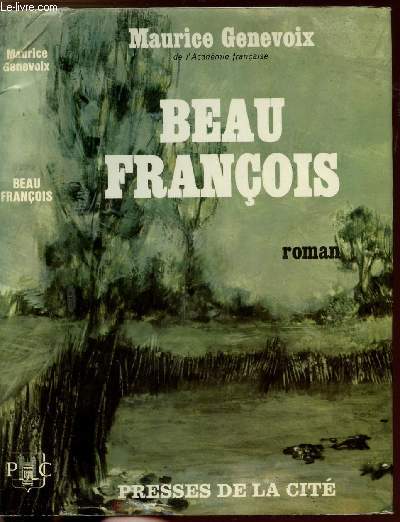This vertically aligned rectangular image is likely a book cover, set against a blurred outdoor nature background with a greenish-gray hue, mimicking the top of the sky fading into tree-covered wilderness and swamp-like water below. At the very top of the cover, in small white letters, it says LE-LIVRE.com. Prominently, the author's name "Maurice Genevoix" (spelled G-E-N-E-V-O-I-X) appears in bold white letters. Centered below, the book's title "Beau François" (spelled B-E-A-U F-R-A-N-C-O-I-S) is displayed in large, all-caps bold white letters. Slightly to the right of the title, smaller black text reads "Roman" in lowercase. Finally, at the very bottom, in all-caps white letters, it states "Presses de la CITE." The overall color scheme is dark, with shades reminiscent of army green, giving the cover a somber and natural aesthetic.